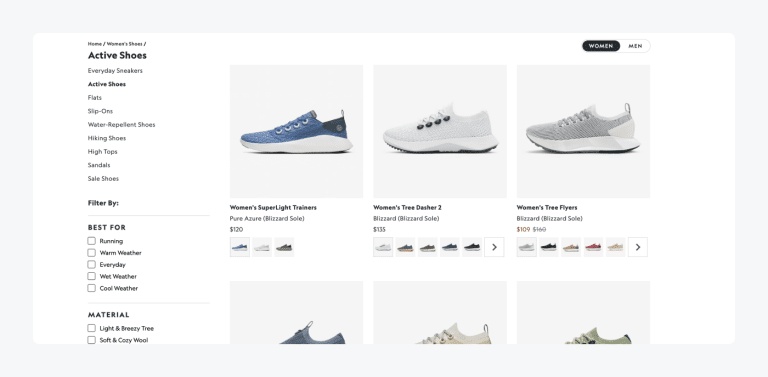This image depicts a webpage from a shoe retail website. The background of the webpage is a light gray color, while the inner section where the content is displayed is white. At the top of this page, there is a navigation menu with options including "Home," "Women's Shoes," and "Active Shoes." The "Active Shoes" category is highlighted and appears larger, indicating it is the currently selected section.

Beneath the main navigation, there are additional categories such as "Flats," "Slip-ons," "Water Repellent Shoes," "Hiking Shoes," "High Tops," "Sandals," and "Sale Shoes." These categories are listed vertically down the left side of the page. There is also a "Filter By" section allowing users to further refine their search based on specific criteria. Under "Best For," users can choose among options like "Running," "Warm Weather," "Everyday," "Wet Weather," and "Cool Weather." Below this, there is a section labeled "Material," where users can filter by "Light and Breezy Tree" or "Soft and Cozy Wool."

In the central area of the webpage, there are images of various shoes from the active shoe category. Each image displays a single shoe, along with options below it to view the shoe in different colors. The price of each shoe is also indicated. However, the bottom row of the webpage is partially cut off, leaving some details incomplete.